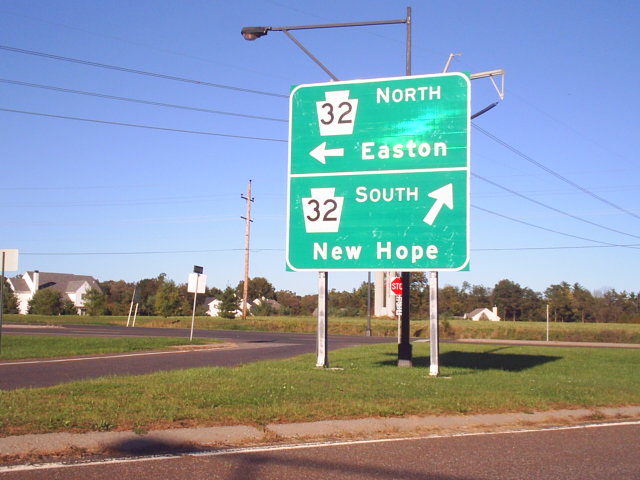The photograph captures a rural intersection marked by a prominent green road sign with a white border, divided into two sections. The top half directs drivers to Northeastern destinations, pointing left towards Easton via Highway 32. The bottom half guides travelers southward to New Hope, with an arrow angled up to the right, also via Highway 32. The scene includes a red stop sign at the intersection, a grassy lot, and a street lamp positioned just behind the road sign. Power lines hang in the sky above, supported by electrical posts. In the background, a clear blue sky stretches over a tree line, behind which several houses are partially visible. The image also shows parts of the horizontal road crossing the lower third of the photo, connecting with a perpendicular road coming from the bottom left. The setting combines elements of rural tranquility with essential directional signage.